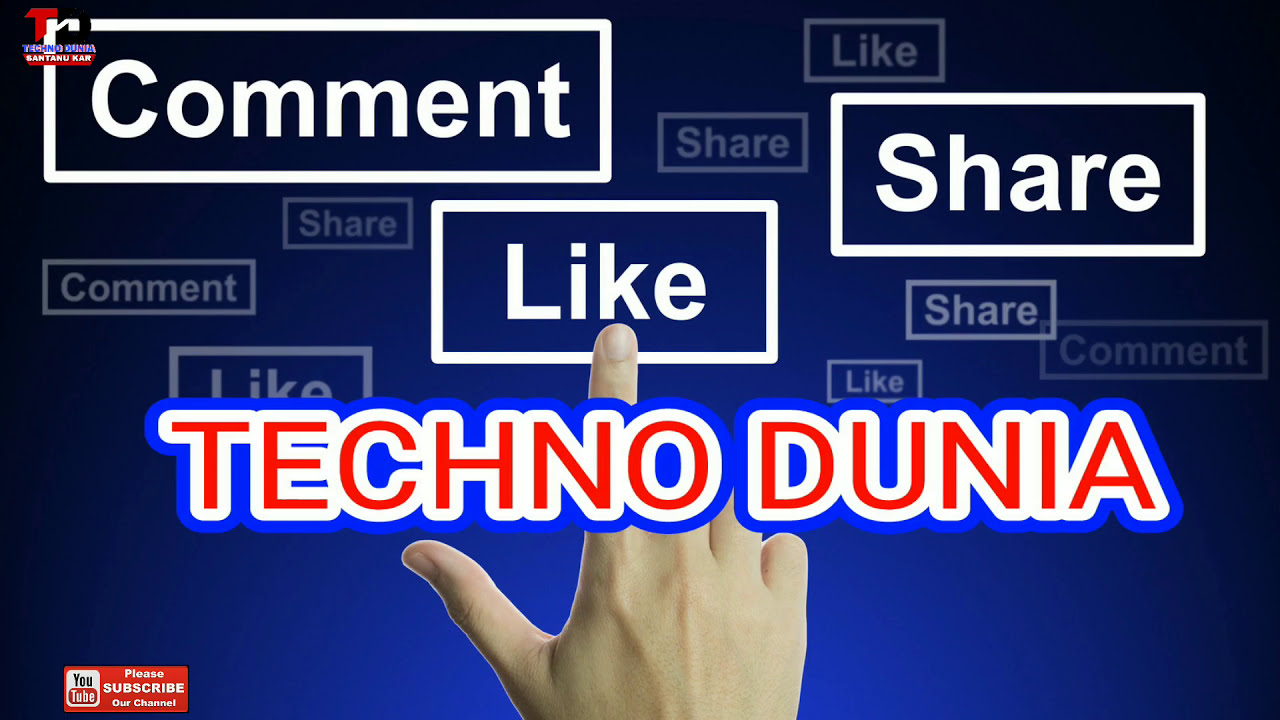The image depicts a YouTube channel page with a dark blue background that transitions to a lighter blue at the bottom. Prominently featured in the center is a hand with its index finger pointing upward, poised as if to interact with the screen. Surrounding the hand are three white rectangular buttons bearing the words "Comment," "Like," and "Share" respectively. These buttons stand out amid numerous dimmer, grayish boxes that repeat the same words in the background. Centrally located on the screen in bold red text is the channel name "Techno Dunia." Additionally, the bottom left corner features the YouTube logo accompanied by the text, "Please subscribe to our channel," in a small red box, confirming that this is indeed a YouTube page inviting user engagement.